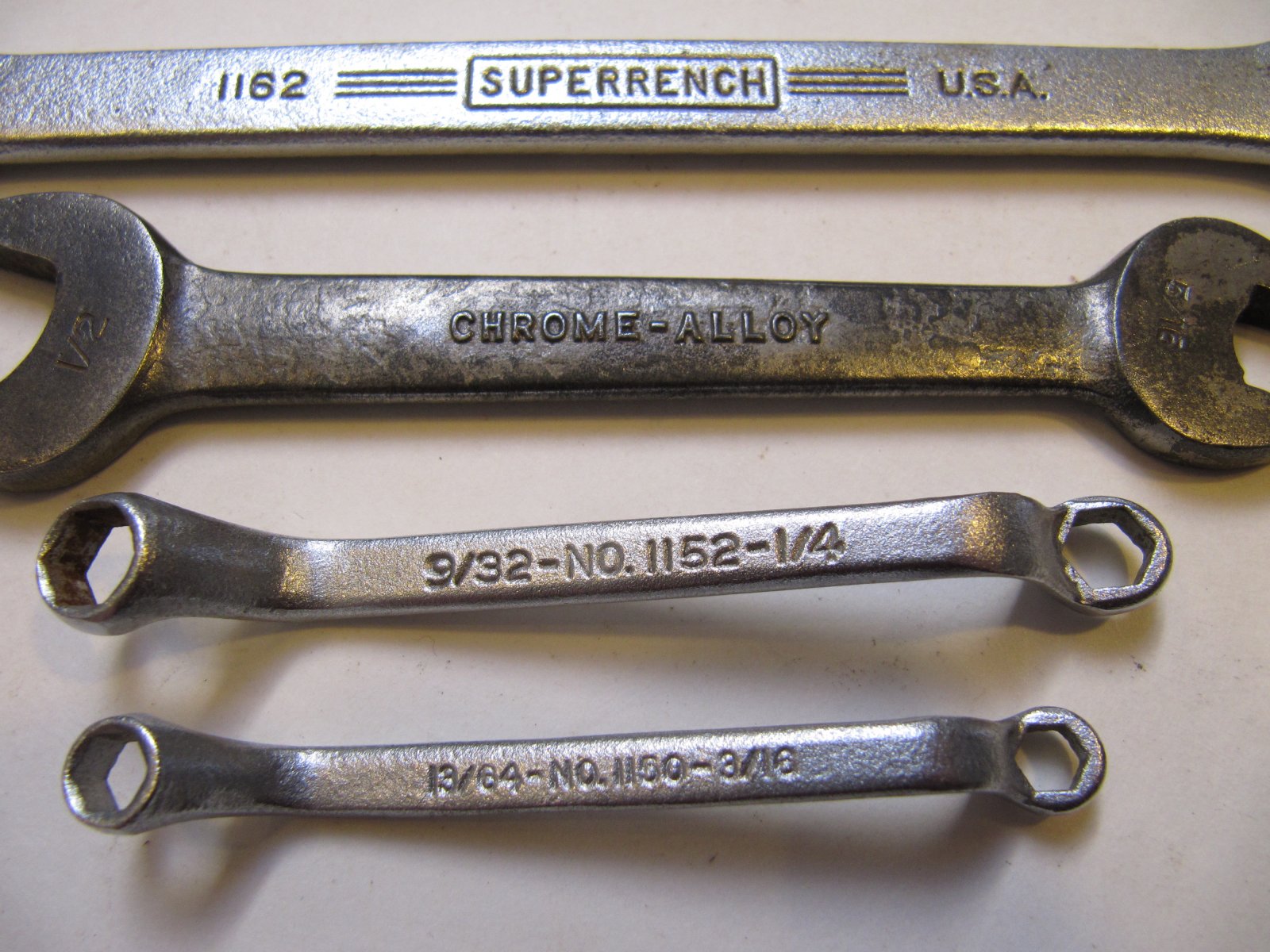The photograph depicts a set of well-used, old wrenches laid out horizontally on an off-white background. At the top of the image, a long, silver wrench stretches across, inscribed with "1162" followed by three horizontal lines, the words "Super Wrench," another set of three horizontal lines, and "USA." Beneath this, a slightly tarnished, darker silver wrench is visible, marked with "Chrome Alloy." The next wrench down is smaller, with circular openings at each end, labeled "932s, number 1152, one quarter." At the bottom of the image, the smallest wrench is positioned, featuring two openings and inscribed with "1364s, number 1150, three sixteenths." The wrenches decrease in size from top to bottom, suggesting their arrangement by length. The photograph is taken from a top-down perspective.